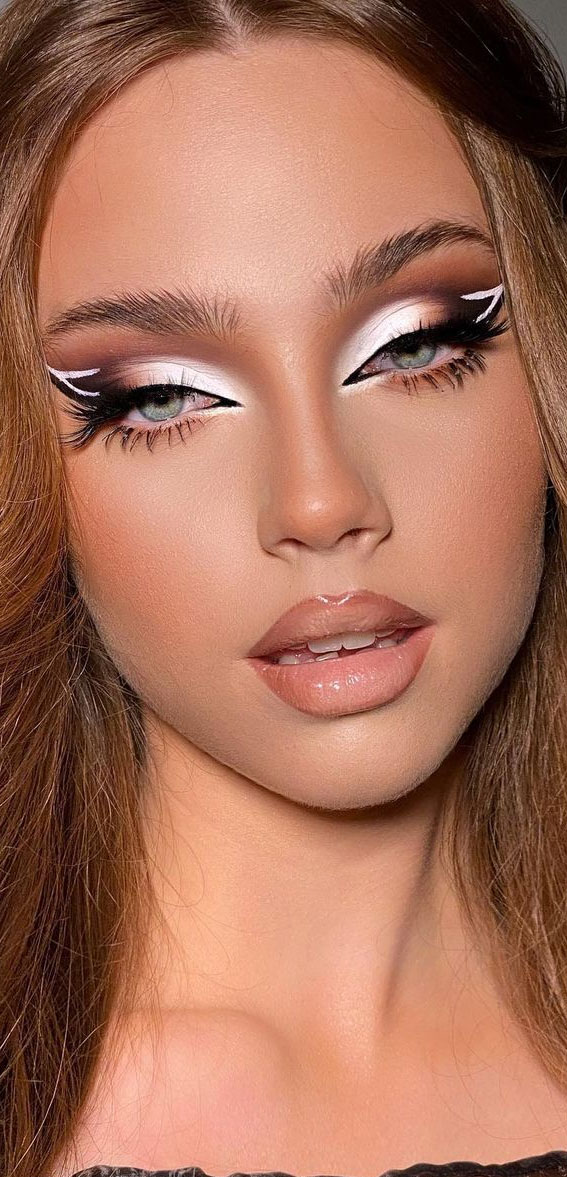This is a close-up professional photograph of a young woman, likely in her 20s, showcasing a meticulously styled appearance. She has long, light brown hair parted in the middle, framing her oval-shaped, light-skinned face. Her makeup is heavily applied in an artistic, Instagram-influencer style, with an emphasis on her eyes and lips.

Her eyebrows are dark brown, well-groomed, and fluffy. She wears dramatic eye makeup that features a gradient of eyeshadow: white in the inner corners transitioning to warmer beige and brown shades towards the outer edges. This is accompanied by intricate black winged eyeliner, accentuated with white liner creating a 'cat eye' effect, notable for the sharp white 'V' shapes at the inner corners. Her eyes are blue or possibly greenish-gray, adorned with thick, long black false eyelashes on both the top and bottom.

Her lips are over-lined with a nude mauve color, filled in with a peachy or light pink glossy lipstick. Her mouth is slightly open, revealing a glimpse of her teeth. Below her neck, a dark-colored top—likely black—is just visible. Her overall look is enhanced by a smooth complexion with a hint of blush, giving her skin an almost flawless appearance.

The image captures her from just below the neck to the top of her head, emphasizing her symmetrical features and polished makeup, making it a striking representation of contemporary beauty standards.